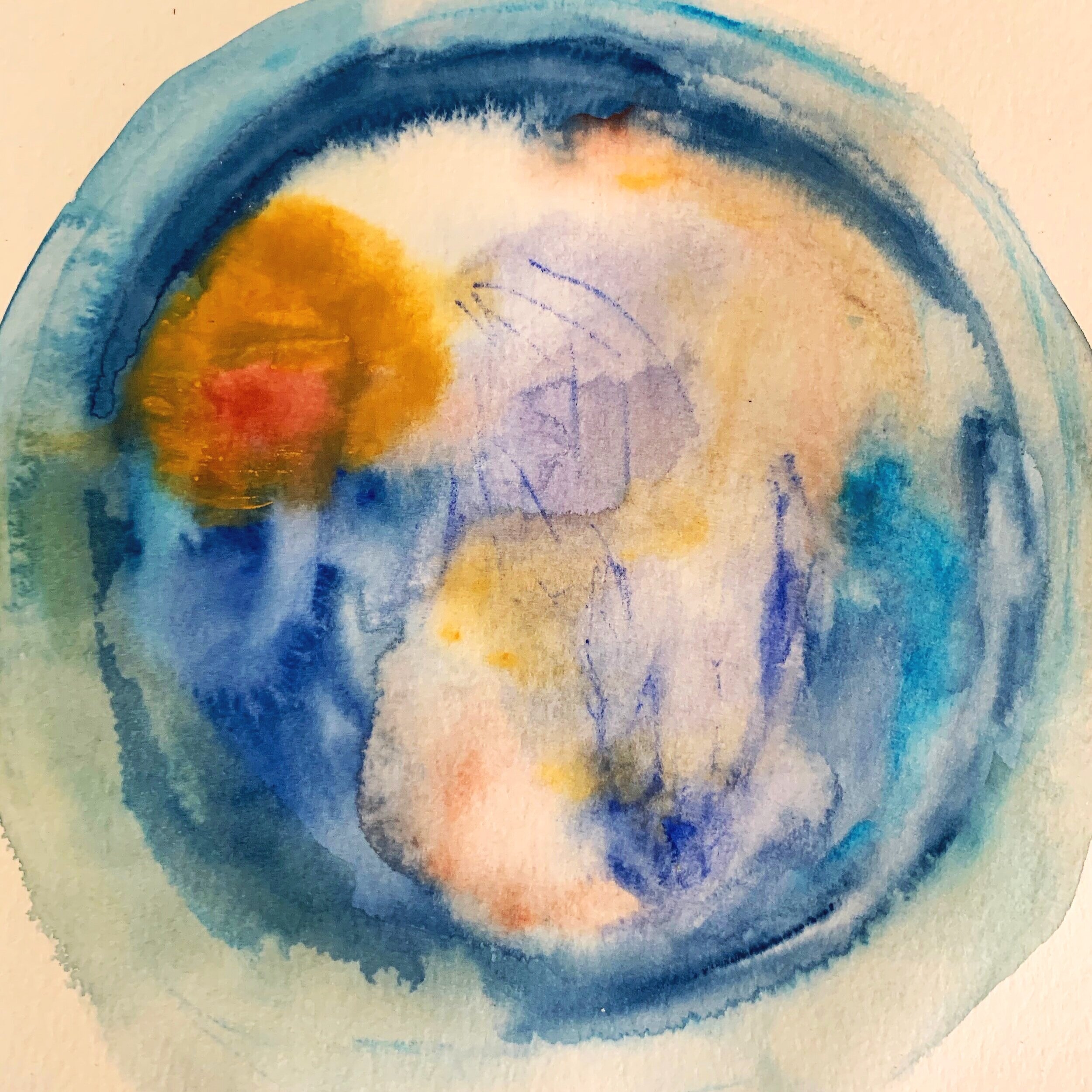This image is a square-format, abstract watercolor painting titled "Earth Dreams" by Amy Kisei. It features an irregularly shaped circle set against a cream background. The circle is primarily composed of a light blue wash interspersed with transparent aqua hues. At the top of the circle, a darker blue ring fades into a series of splashes in bright blue and gold on the left side. Within the inner portion of the circle, a sketchy purple figure appears, complemented by a gold wash that gradually transitions into a bluish wash below it. The painting also includes subtle hints of teal and orange, contributing to its complex, modern aesthetic. The overall impression suggests a conceptual exploration, potentially evoking images of the Earth.